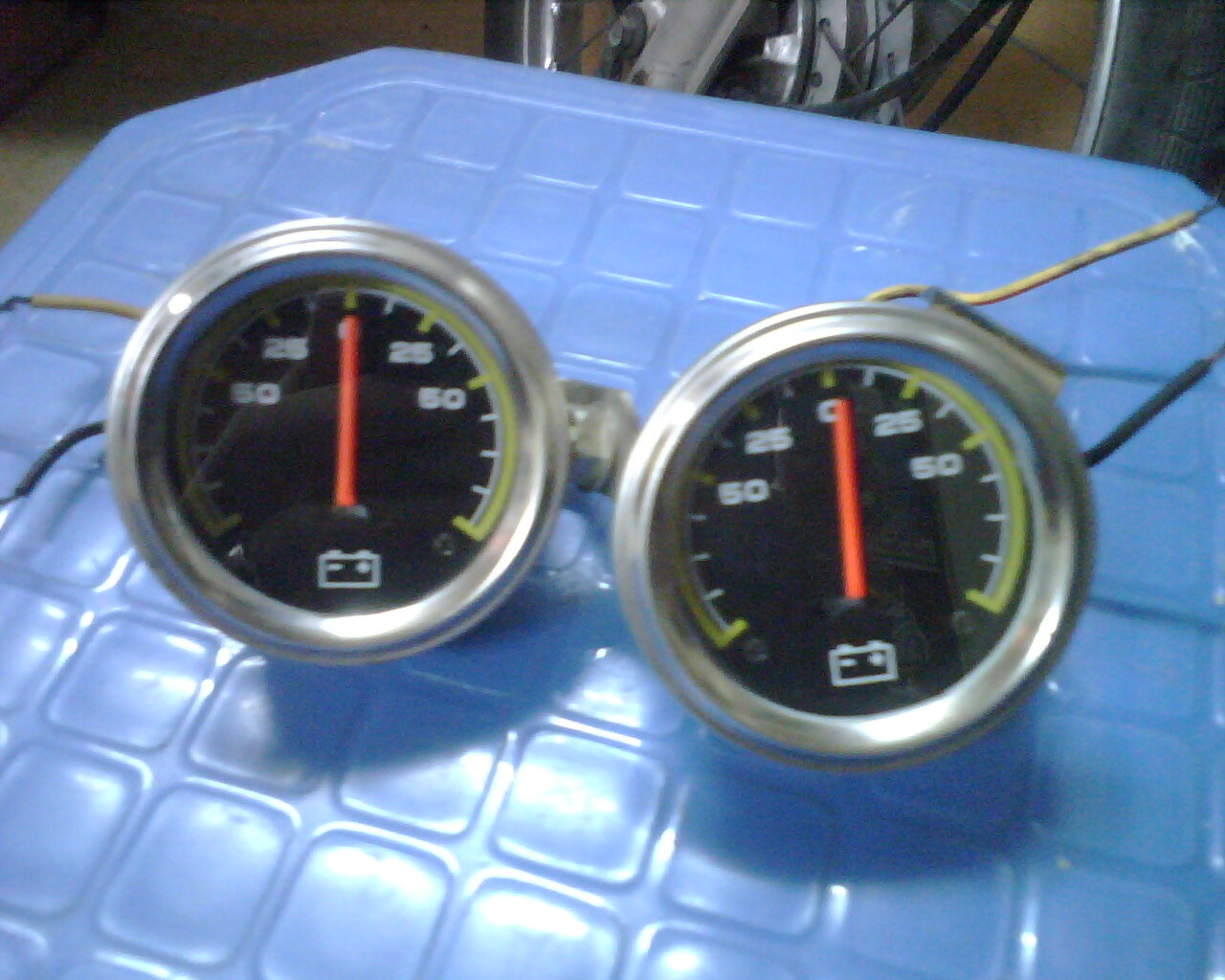This photograph captures two identical gauges, likely designed for a motorcycle, given their size and structure. Each gauge is circular with a metallic silver ring encasing a black face. Prominently featured on the face is a long orange needle, bordered by a yellow scale with hatch marks. The top of the scale is marked as zero, with 25 indicated on both the left and right, and 50 located approximately at the 10 and 2 o'clock positions. A white battery icon with a minus and plus symbol is visible at the bottom of each gauge, suggesting that these meters likely measure electrical charge or battery health. The gauges are positioned on a small, blue plastic tray within a garage setting. In the backdrop, part of a motorcycle wheel is faintly visible at the upper edge of the image, reinforcing the assumption that these gauges pertain to a motorcycle.